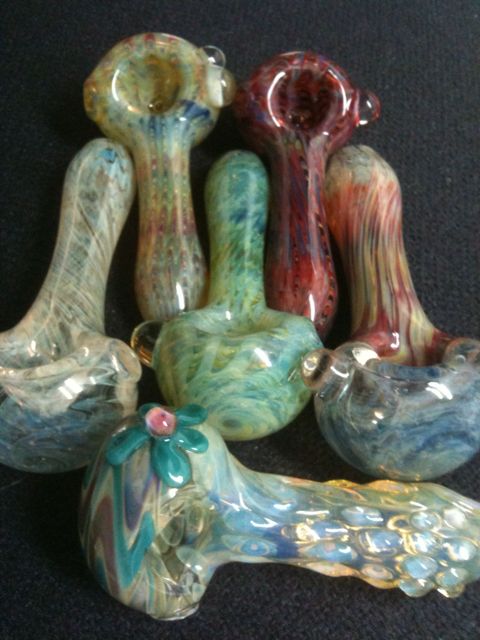The image showcases six colorful, hand-blown glass pipes arranged on a dark, cloth-like background. The bottommost pipe is horizontally oriented, featuring a bulbous left end with a blue flower and a pink center, and a bumpy protrusion extending to the right. This pipe displays a palette of blue, yellow, and clear glass. Positioned above it are five vertically oriented pipes. The three on the left exhibit primarily blue-green hues with one of them containing varied colors including blue and red. The fourth pipe is mostly red with accents of purple, while the fifth is a mix of white, beige, and blue. Each pipe combines a rounded end, resembling a bowl, and a stem that appears slightly indented like traditional smoking devices. The vivid color variations and delicate craftsmanship highlight the artistry of these glass creations.